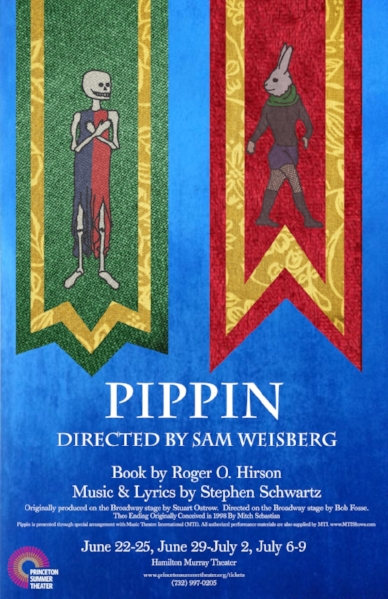This is a detailed poster for the play "Pippin," directed by Sam Weisberg. The background is a striking blue, adorned with two vertically hanging ribbons. The left ribbon is green with gold interlay, featuring a skeleton clad in a robe divided into blue on the left and red on the right, with its arms crossed over its chest. The right ribbon is red with gold interlay, showcasing a human figure with the head of a rabbit, dressed in a green scarf, brown shirt, purple skirt, and boots. Below the imagery, the text in white reads "Pippin, directed by Sam Weisberg, book by Roger O'Hurston, music and lyrics by Stephen Schwartz." The poster details specific show dates: June 22nd-25th, June 29th-July 2nd, and July 6th-9th, and the location as Hamilton Murray Theater, with a contact phone number provided at the bottom. This eye-catching design serves as an advertisement for the theatrical performance.